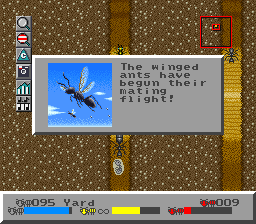This is a detailed screenshot from a vintage computer game, likely from the late 80s or early 90s, marked by its pixelated graphics. The image has a square shape with symmetrical sides. The bottom section of the screenshot features the game’s UI, consisting of a gray banner running horizontally across with three distinct bars. The first bar on the left showcases a picture of a blue bee accompanied by a blue bar, indicating a form of meter or status. Next to it is a yellow bee with an infinity symbol next to a yellow bar, and the final bar depicts a red bee with a corresponding red bar. Central to this image is a large gray rectangle displaying an illustration of black winged ants in flight, with black text declaring, "The winged ants have begun their mating flight." The backdrop reveals a network of tunnels populated by crawling ants, transitioning in color from brown to gold, enhancing the sense of depth and pathway delineation. The background is predominantly brown with white dots, further portraying an earthy terrain. Scattered along the left side are clickable icons or menu items, providing interaction points for gameplay.